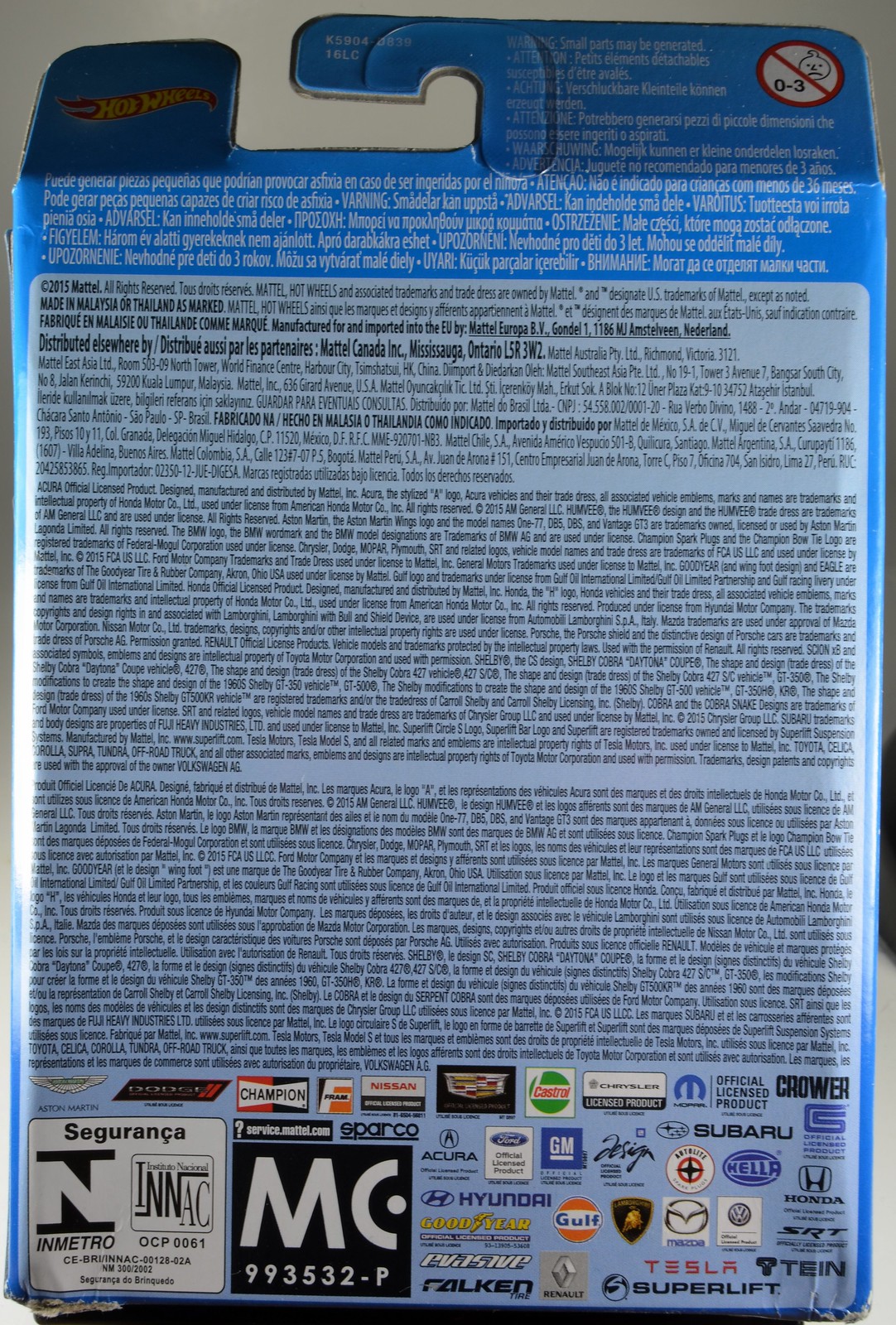The image depicts the back of a Hot Wheels car package. Dominated by a blue background, the upper left-hand corner prominently displays the iconic Hot Wheels logo in yellow set against a red banner. In the top right corner, a warning symbol featuring a baby face with a red circle and diagonal line indicates that the product is not suitable for children aged zero to three years. The packaging is covered in text blocks, primarily detailing safety warnings and product information in multiple languages including English, Spanish, and Russian. A significant portion of the lower half is dedicated to various company logos like MC, Champion, Nissan, GM, Acura, Hyundai, Goodyear, Gulf, Subaru, Tesla, and Honda. Notable details include a copyright notice stating "©2015 Mattel, all rights reserved." The bottom part also features the code "MC993532-P" and the word "Sigurens" amidst the multilingual text. The overall design includes a lighter blue area highlighting the black text for better readability.